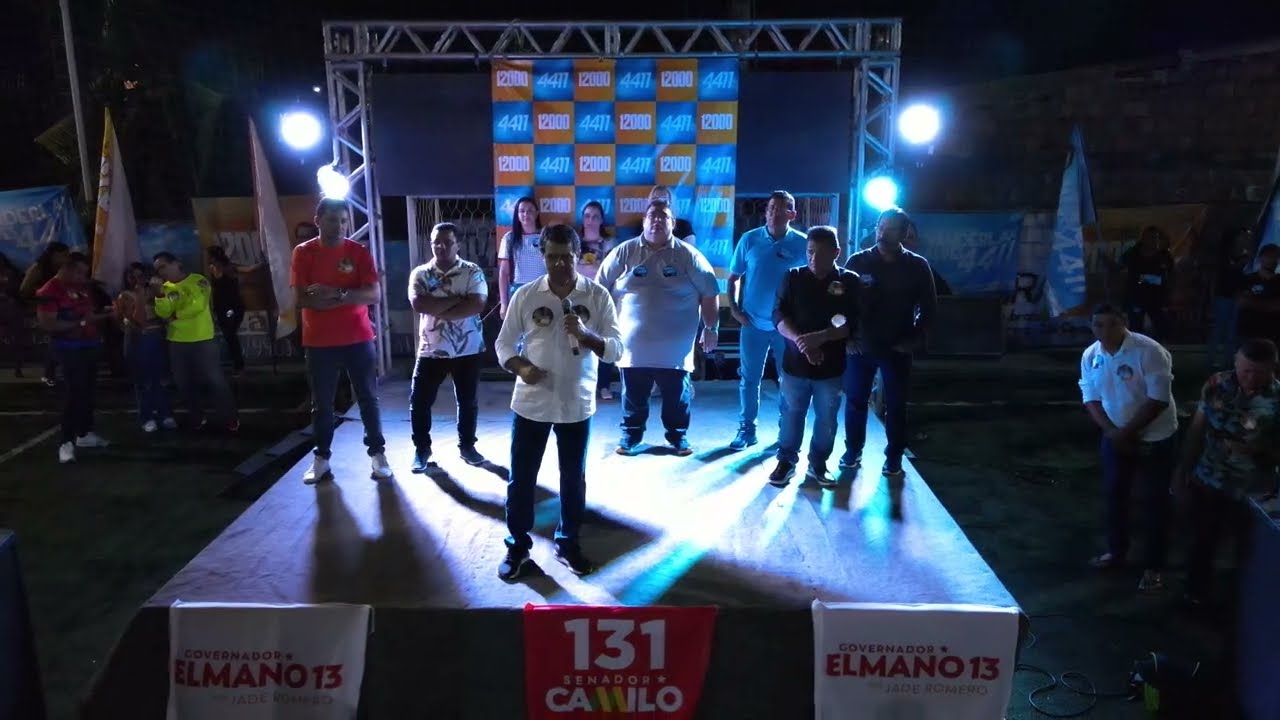The image depicts a nighttime scene on a modestly constructed wooden stage, brightly illuminated by three lights mounted behind it. Nine individuals are positioned in a staggered manner on the stage, including both men and women, with seven men prominently visible and three women towards the back. A man stands front and center, donning a white collared button-down shirt and holding a microphone. The backdrop features a checkerboard banner alternating between orange and blue squares, each containing numbers. The front of the stage is adorned with three banners, displaying slogans and numbers in red and white. From left to right, the banners read “Governado Elmano 13” and “131 Sen. Camillo.” Flags are visible on either side off-stage, contributing to a political rally or public event atmosphere. The stage setup includes a small structure supporting lights and additional materials, casting a bright glow on the participants while the surroundings remain relatively dark.